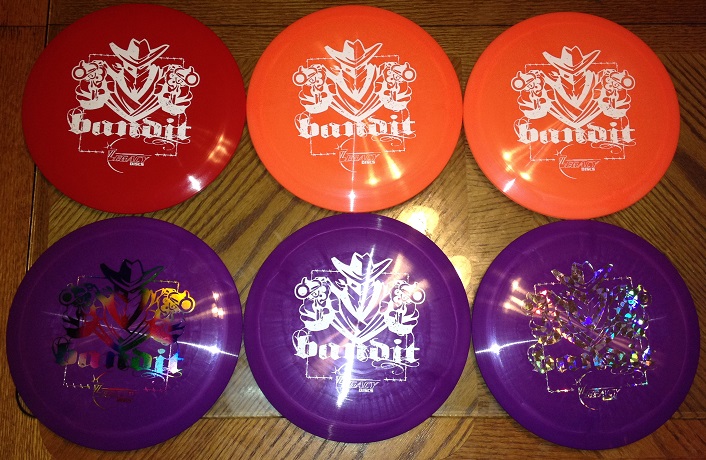This is a detailed photograph of six Frisbee discs arranged on a light-colored, polished wooden table. The table's surface reflects the light, adding an extra shine to the scene. The Frisbees are organized in two columns, with three discs in each. The left column features three purple Frisbees, each adorned with the same logo: a cartoon bandit wearing a cowboy hat and bandana while pointing two guns forward. The logo includes the word "Bandit" in lowercase letters just below the bandit's elbows. The right column has a similar design but different colors: the top disc is red, and the two below it are orange. Each of these Frisbees also bears the 'Bandit' logo, consistent with the ones on the purple discs. Some Frisbees have the logo in a holographic or metallic finish, reflecting multiple colors. The main colors present in the design and reflections include red, orange, purple, white, black, yellow, blue, and green.